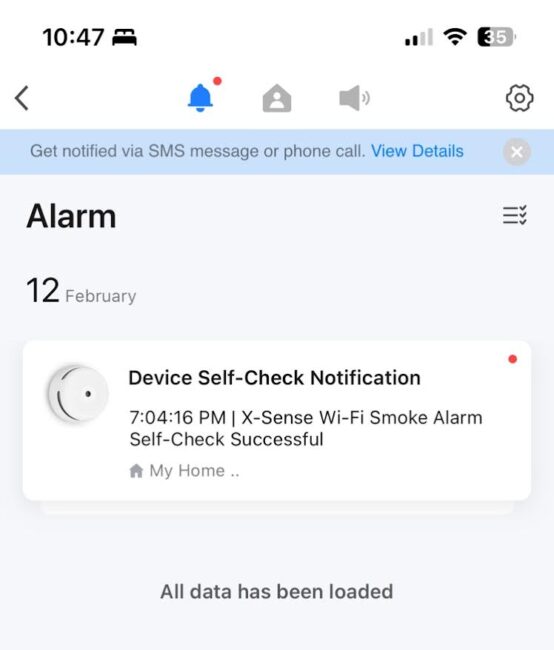This vertical image appears to be a screenshot from a smartphone or similar smart device. Overlaying a plain white background, the interface provides various status icons at the top of the screen. On the left side, it displays the time as "10:47" in bold block text, coupled with a small icon. To the right, indicators show the signal bar strength, Wi-Fi connectivity, and a battery level at 35%.

Directly below on the left, there’s an arrow icon followed by a highlighted blue bell icon, indicating notifications. Adjacent to this, in gray, are icons for a home (represented by a small house with a person inside), volume control settings, and a general settings gear icon, spaced out across to the right.

A light blue strip runs horizontally, suggesting an alert with the text, "Get notified via SMS message or phone call," followed by "details" in blue and a gray circle with a white "X" for dismissal.

Below this alert, a gray section organizes the main content. At the top in bold block letters, it reads "ALARM," followed by the date "12th of February." Central to this section is an image of an alarm device with the accompanying text: "Device self-check notification, 7:04:16 PM, XSENSE Wi-Fi smoke alarm, self-check successful, My Home."

At the bottom of the gray section, the text concludes with "All data has been loaded. Awesome alarm."

On the far right side are three horizontal lines, each with a check mark next to it, possibly indicating a checklist or steps completed.